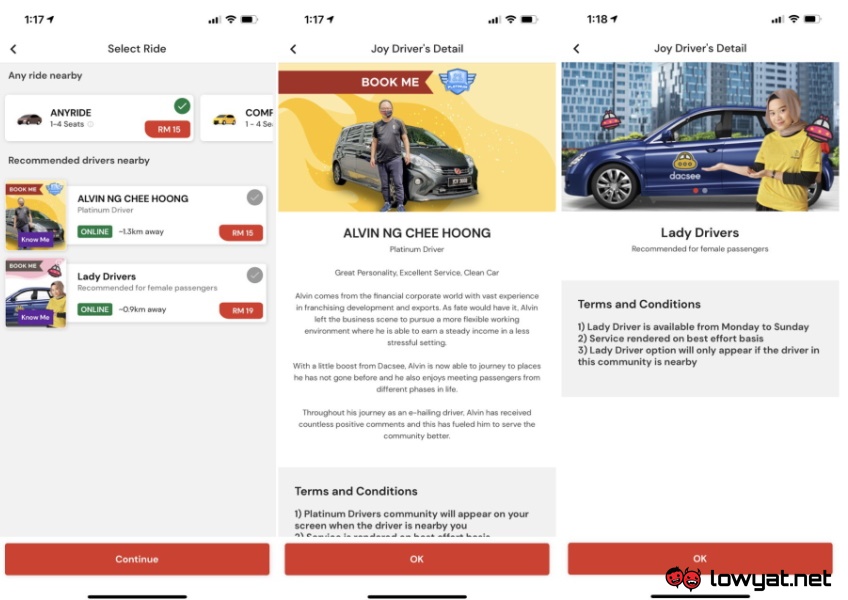This detailed and organized caption accurately represents the content and layout of the screenshot:

---
The screenshot is divided into three primary rows of information, each packed with details. At the very top, a set of numeric times “1:17, 1:17, 1:18” is displayed alongside battery icons and signal strength indicators.

Below this top section, the first row is titled "Select Ride" and contains three entries labeled "Joy Driver Seatail" across it. 

The second row features three columns. The left column, titled "Any Ride Nearby", includes small images. The middle column, labeled "Book Me", showcases an image of a black vehicle with a man standing in front of it against an orange background. This person is identified as Alvin NGCHEE HOONG, a Platinum Driver. 

The third column, also labeled "Joy Driver Seatail", displays a blue car positioned in front of high-rise buildings. In the foreground, a woman dressed in an orange shirt and wearing a brown scarf stands with her hands outstretched, emphasizing the car. This section includes a note reading "Lady Drivers, recommended for female passengers" and a mention of "Terms and Conditions".

Under these three rows, at the bottom, are three red bars labeled "Continue", "OK", and "OK". The entire page ends with the web address "toyat.net”.
---